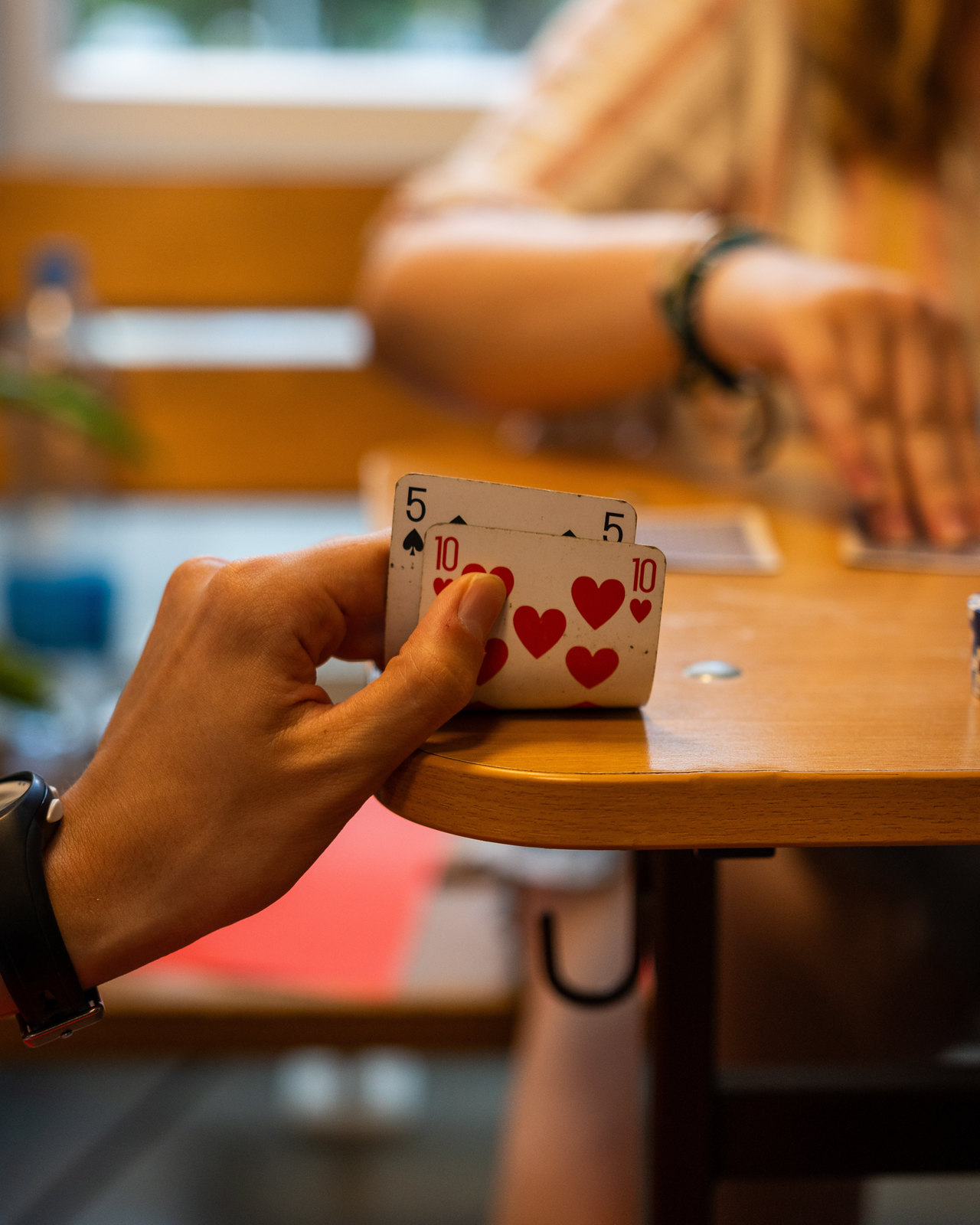In this vibrant color image, two individuals are engaged in an intense game of cards at a wooden table. From the left edge near the bottom of the photograph, a hand adorned with a black watch—a portion of its face cropped by the photo's edge—emerges into the frame. The hand delicately grasps two playing cards between the forefinger and thumb, the cards' tops bent upward, revealing a 10 of Hearts (in vivid red) and a partially visible 5 of Clubs (in striking black).

In the background, to the top right of the scene, another figure is slightly blurred. This person, wearing a short-sleeved striped shirt, extends their right arm and carefully touches a playing card on the table with two fingers. The face of this card is hidden from view as it rests facedown. An adjacent playing card lies to the left of it.

The backdrop features a wall and the edge of a window framed with white trim, all softly blurred to focus attention on the card game. The background figure’s chest, upper arm, and a hint of their hair are faintly discernible through the blur. The meticulous detail captures the intensity and concentration of the players, situating the viewer at the heart of the game.